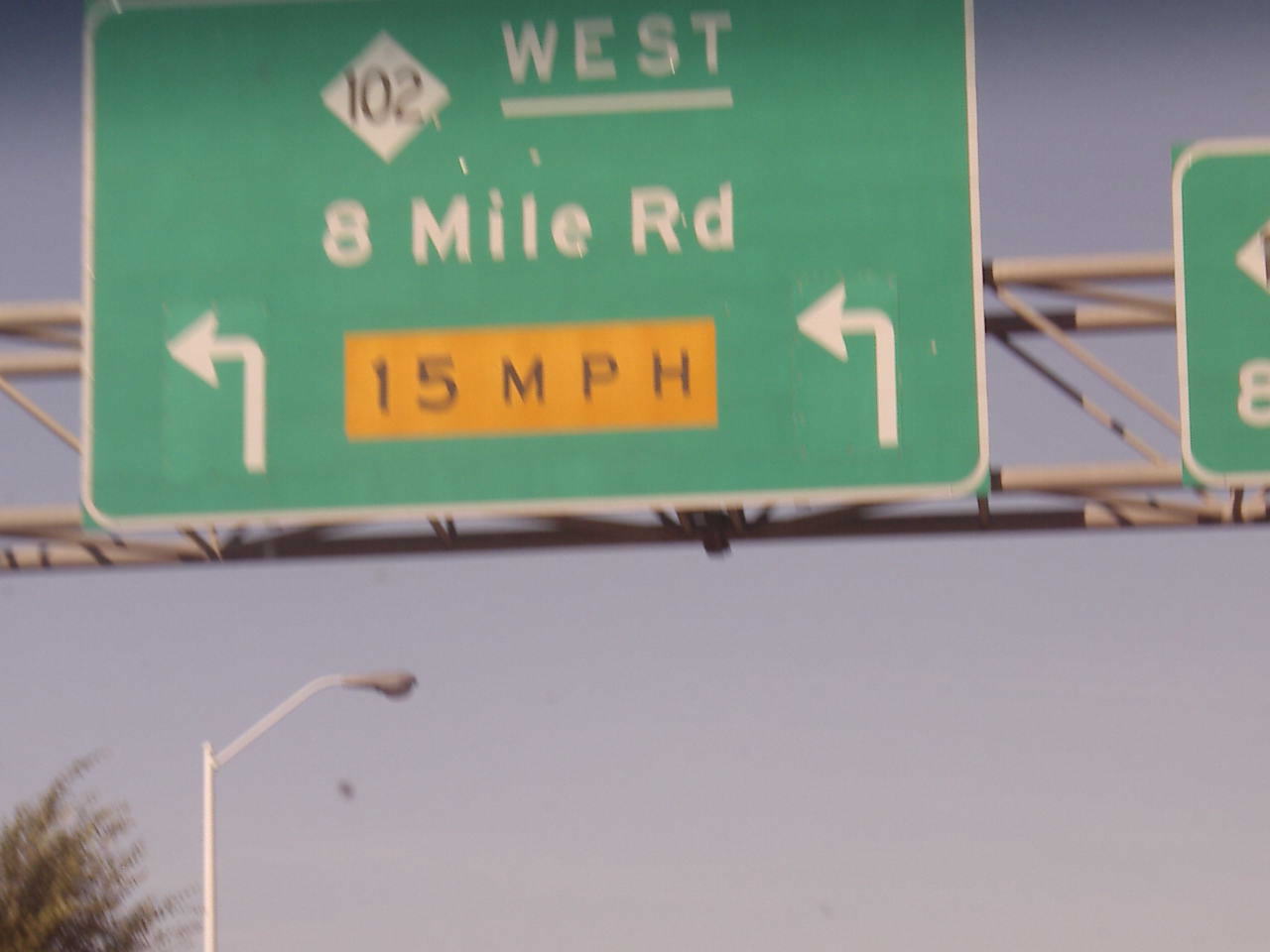In this image, we are looking up at a large green highway sign mounted on a metal structure, possibly above a road or motorway. Against the backdrop of a purple-blue sky, the sign prominently displays the numbers "102" inside a white diamond, followed by the text "West" in white, underlined. Below this, in bold white text, it states "8 Mile Road". Beneath these words, a long yellow rectangle features the indication "15 MPH" in black letters, flanked by two white arrows pointing left. To the side, only a portion of another green sign is visible, showing the number "8" and a left-pointing arrow. In the lower left corner of the image, a street lamp with an angled white pole and what appears to be a bush or tree is visible. The signs and lamp are mounted on a complex, scaffold-like structure of tubes and brackets.